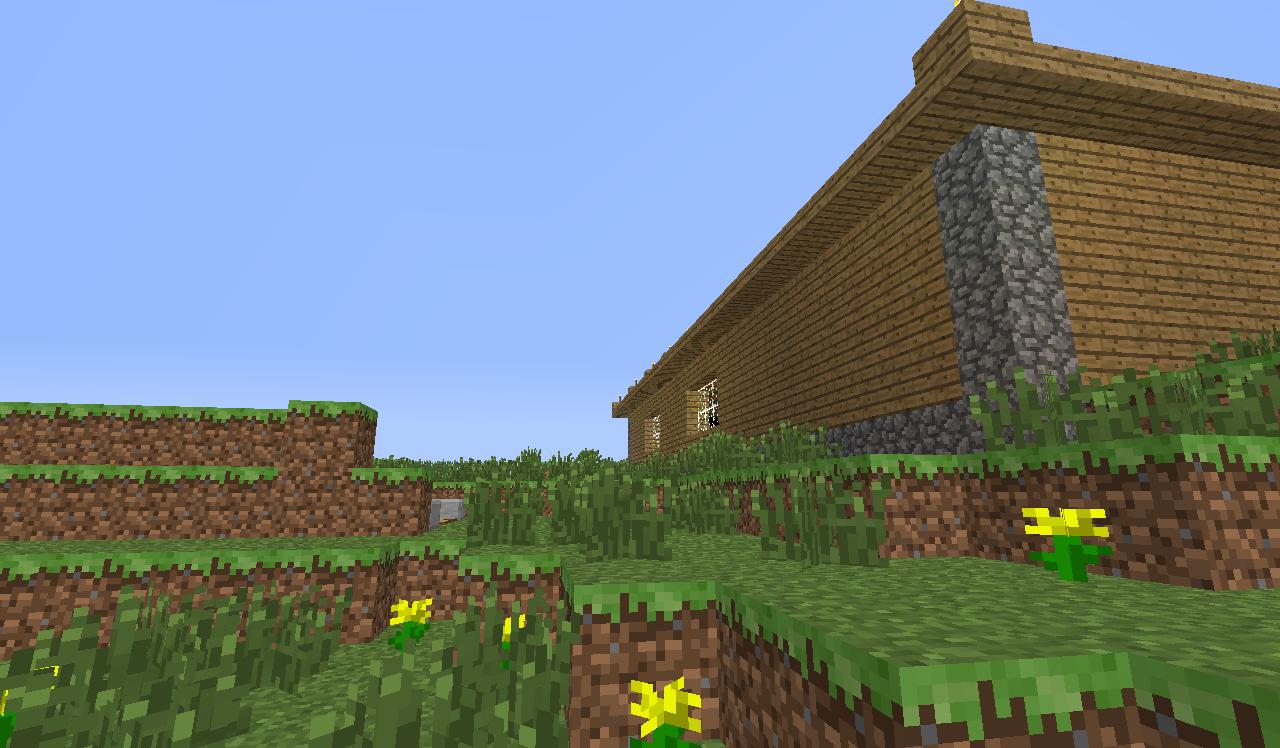The image resembles a scene from a video game, artfully constructed with multicolored blocks. It features a single-story home with brown wood paneling and stone corners made of gray blocks. Surrounding the house is neatly arranged landscaping, including well-placed bushes and a low brick wall that encircles the property. The terrain then steps down to a lush, green lawn dotted with bright yellow flowers. The scene further extends to a cliff edge, where the grass abruptly transitions into an exposed layer of earthy brown soil. The entire setting exudes a pixelated charm, reminiscent of classic block-style video games.